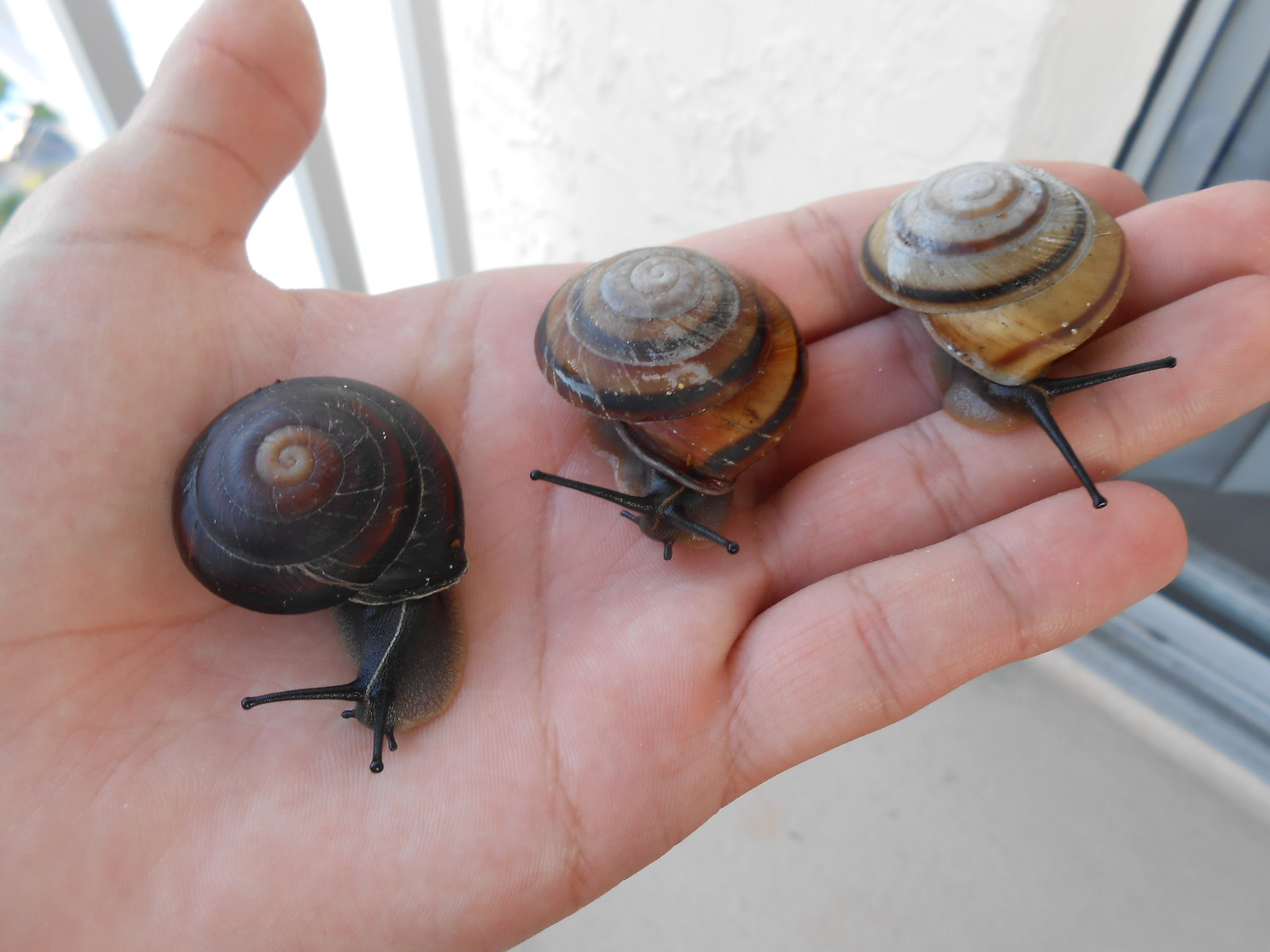This photograph is a detailed close-up of a man's left hand, palm facing upward, holding three snails. The setting is outdoors, likely in the shade, with a sliding glass door and a pale grey frame visible on the right side of the image, while the ground is concrete and the wall above is white. The man's thumb is positioned in the upper left corner of the picture.

In the palm of his hand, three snails are emerging from their spiraled shells, their tiny antennae visible. The first snail, closest to the upper part of his palm, has a dark brown shell with a light tan center and a noticeable spiral pattern. This snail appears to be slightly darker than the others. The middle snail features an amber-colored shell with a black outline forming its spiral, and is in the process of peeking out of its shell. The third snail, near the man's fingertips, boasts a cream pearly shell with red and brown markings along its spiral, with just its head and feelers extending out. All three snails appear to have black bodies. The overall composition captures the delicate beauty and distinct shell patterns of each snail.